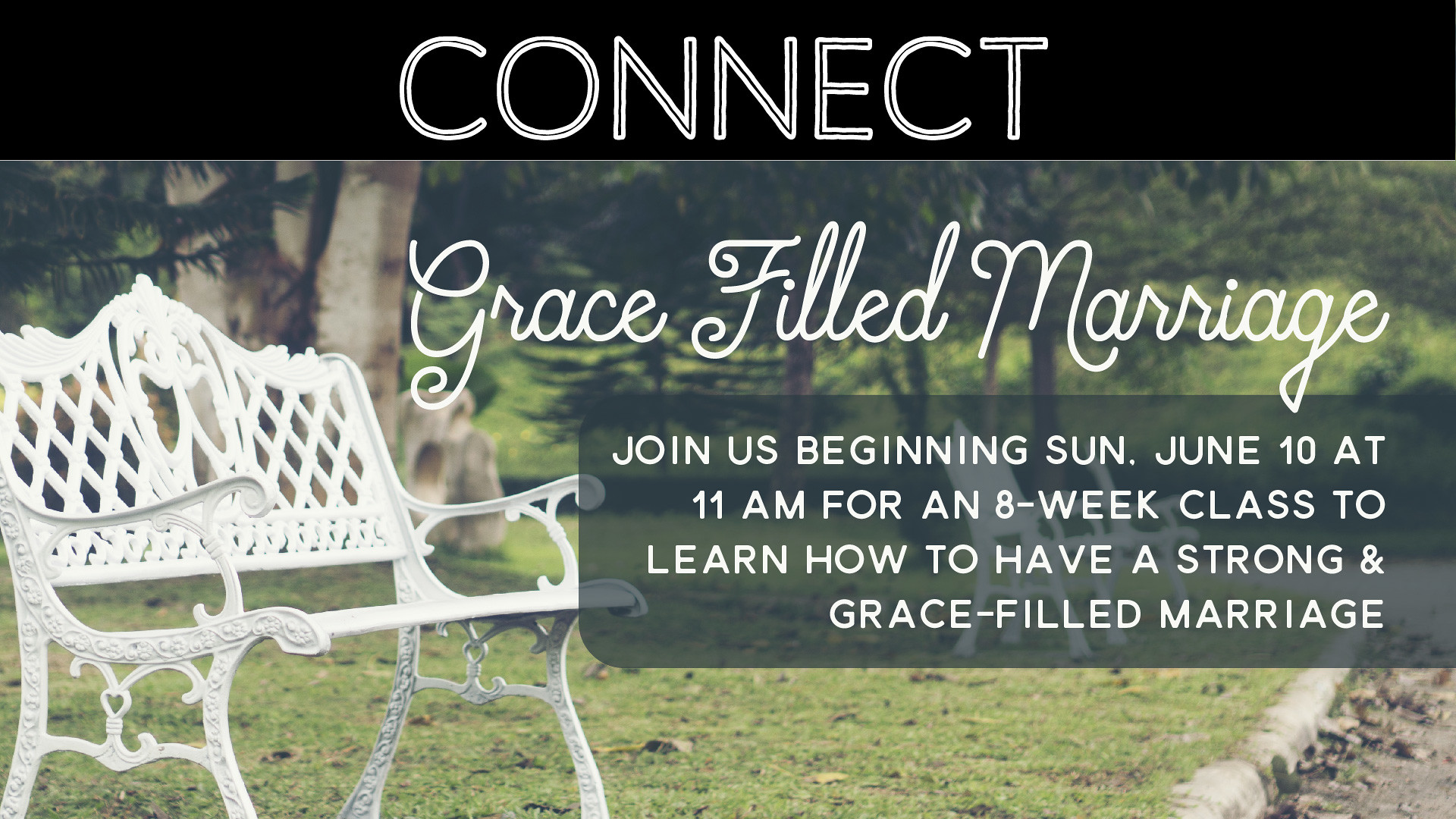The image is an advertisement for a course titled "Grace-Filled Marriage." It prominently features the word "CONNECT" in bold, white capital letters over a black ribbon at the top. Below this is the invitation text: "Join us beginning Sunday, June 10 at 11 a.m. for an eight-week class to learn how to have a strong and grace-filled marriage." This text appears in a stylized cursive font within a transparent dark box with rounded edges, nicely contrasting the background. The background depicts a tranquil park scene with a white cast-iron bench featuring an ornate design placed on short grass. Adjacent to the bench, on the left side, stands a tree, and more trees are visible in the distance under a partly blue sky. The image uses a soothing color palette of white, black, green, brown, and blue, evoking a peaceful and inviting setting.